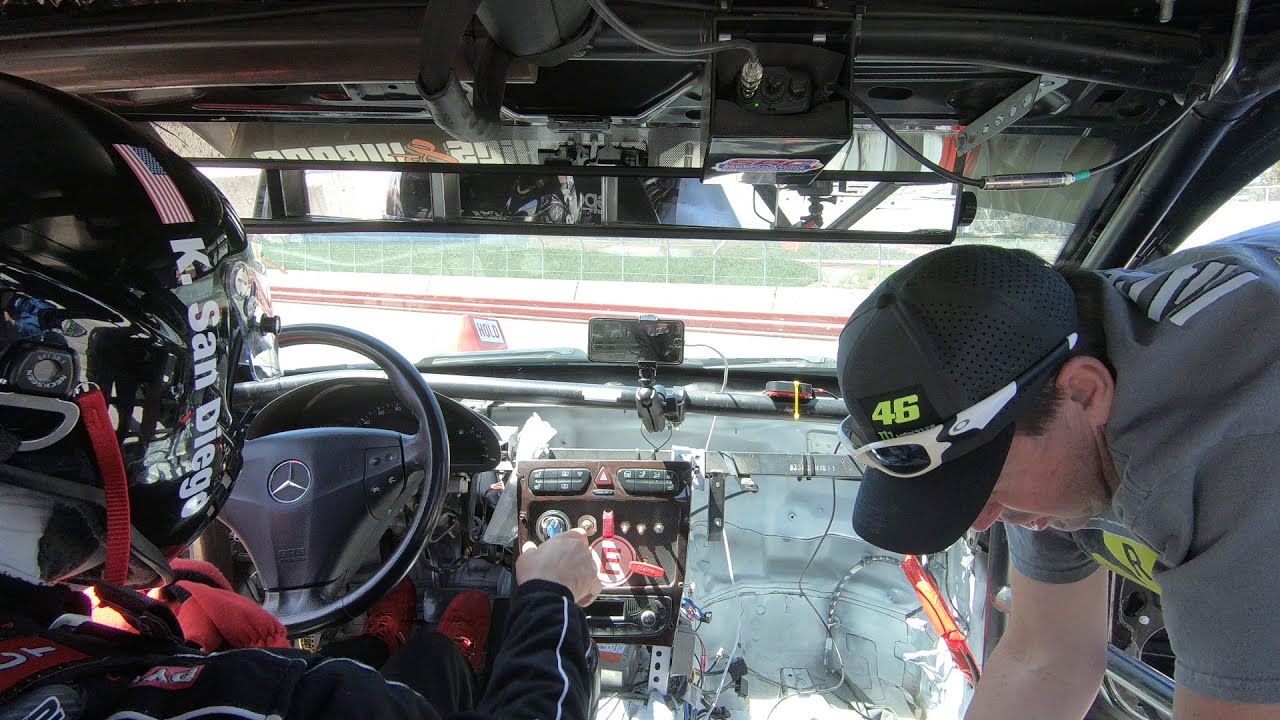The image depicts the interior of a high-performance race car, possibly from a NASCAR or similar racing series. The driver, situated on the left side of the image, is wearing a black helmet adorned with white vertical lettering that reads "K. San Diego" and features an American flag. The driver, clad in a long-sleeved black jacket with white pinstriping, has his hands on the shifter and is wearing red shoes. The race car's steering wheel, which displays the Acura logo, is also visible. On the right-hand side, another man, wearing a short-sleeved gray shirt and a black baseball cap with white sunglasses on the brim, is bending into the car, appearing to check or fix something amidst a tangle of wires and electrical equipment. The car's interior is predominantly black, with a white ceiling, and out the windshield, the race course can be seen, featuring a fence, red stripes on the road, and a red sign that reads "Hold."